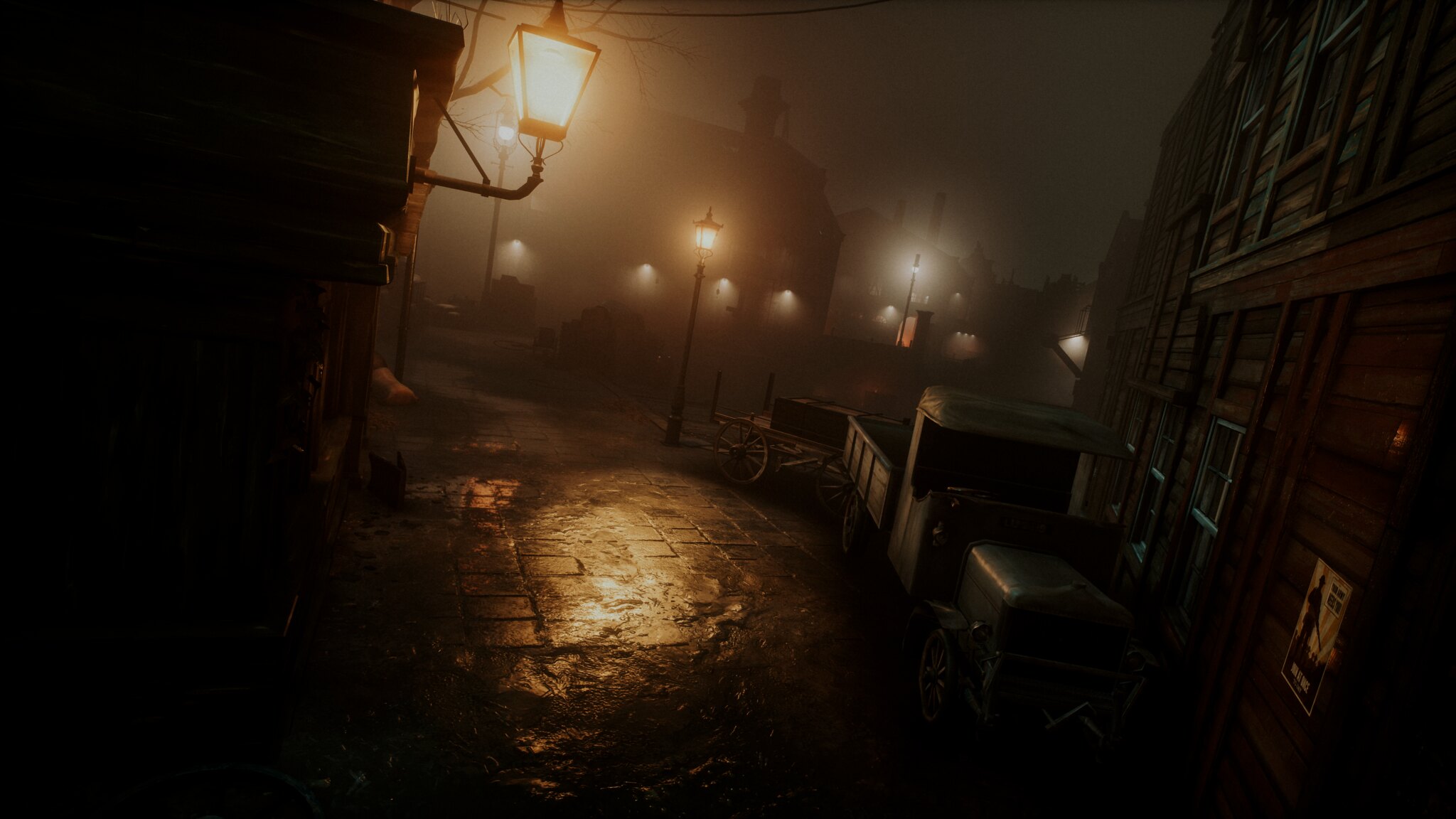In this nighttime video game scene, the setting depicts an outdoor environment. On the left side of the image, there is the edge of a completely black wooden building. This structure features a lantern hanging from a curved pole near the front side, emanating a soft, yellow light. The ground is covered with a cement or paving stone floor, which catches the glow from the lantern. Towards the right, two brown wagons with gray canvas tops, allowing space for passengers, are situated. Further to the right, there is another brown building with a couple of windows, adding to the rustic allure. In the distant background, a tall building stands prominently against the very dark gray night sky, contributing to the atmospheric depth of the scene.